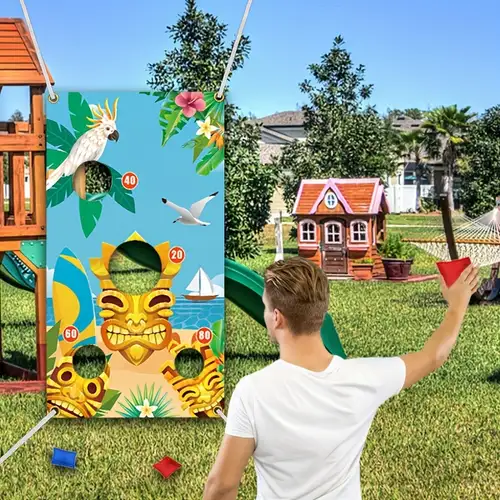In the vibrant outdoor scene, a man in a white t-shirt stands poised to throw a red beanbag as he plays a lively game of cornhole. The cornhole board, adorned with an island party theme, is decorated with tropical birds, pink flowers, white stars, and a majestic sea backdrop featuring a sailboat. The board, elaborately designed with a totem pole displaying a tiki figure with an elongated smile and slanted eyes, has multiple holes for scoring, marked for 20, 40, 60, and 80 points. The largest hole is situated at the top of the totem's head, while two smaller holes lie at the base. This colorful board is set against a green slide of a children’s fort within a playful yard, complete with green and yellow grass, a small child-sized playhouse with an orange-brown roof and three windows, a nearby doghouse, and surrounding trees. Two hacky sacks, one blue and one red, rest on the ground in front of the cornhole board, emphasizing the game's festive and inviting atmosphere. Amidst this joyful setting, the clear blue sky hints at a perfect day for outdoor fun.